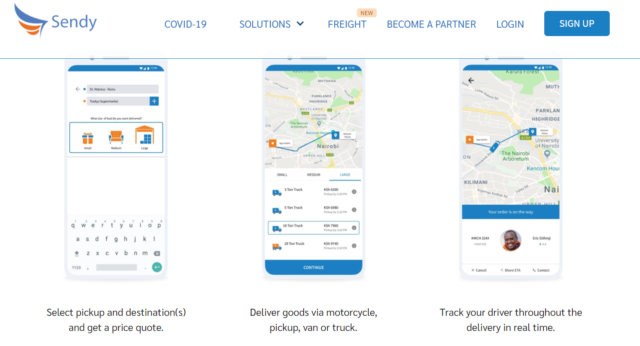In this image, set against a solid white background, we see a detailed layout featuring both visual and textual elements. In the upper left corner, there is a logo adorned in blue and orange, followed by the word "Sendi" in blue text. To the right of the logo, the phrase "COVID-19 solutions" is displayed, accompanied by a pull-down arrow. Next, the word "Freight" appears with a small box labeled "new" alongside it. Further right, the options "Become a partner," "Login," and "Sign up" are clearly listed, with the "Sign up" button highlighted in blue for emphasis.

Beneath these elements are three distinct screenshots. The first screenshot, positioned on the left, includes a small black text caption that reads, "Select pickup and destination and get a price quote." To its right, the second screenshot features a map interface and an accompanying description stating, "Deliver goods via motorcycle pickup, van, or truck." The final screenshot on the far right showcases another map, alongside a color photo of an African-American man. This screenshot is described with the text, "Track your driver throughout the delivery in real time."